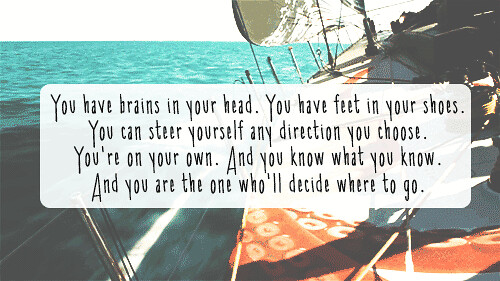The image depicts a sailboat leaning toward the left, navigating through the calm teal waters of the ocean. The boat is painted in a striking blue color, contrasted by its mostly white interior. The scene captures small ripples on the aquamarine water, with the horizon visible in the background where the ocean meets the sky. Central to the image is an overlaid gray, rounded rectangular speech bubble containing an uplifting and inspirational quote in black text: "You have brains in your head. You have feet in your shoes. You can steer yourself any direction you choose. You're on your own, and you know what you know, and you are the one who will decide where to go." This quote, reminiscent of Dr. Seuss's encouraging words, promotes the spirit of adventure and self-determination. The sailboat also features a red octopus tentacle painted on its stand area, adding a touch of uniqueness to the vessel. The interior is equipped with oars and supplies, neatly stored in baskets, ready for the exploration ahead. The overall image evokes a sense of readiness and excitement to take charge of one's own journey.